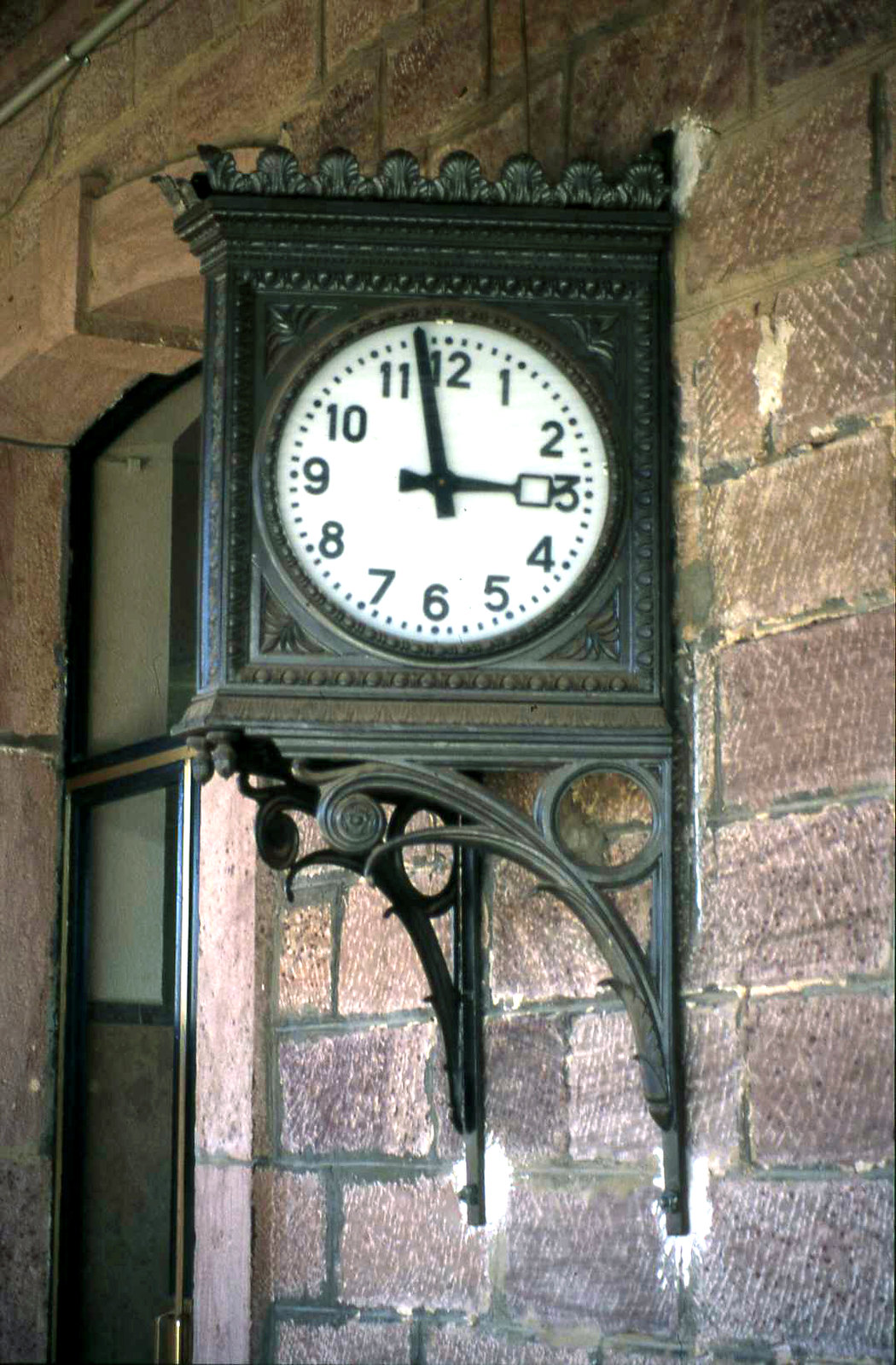This image depicts an intricately designed wall clock, which is mounted on a weathered brick wall characterized by a mixture of purples and darker reds, indicating its age. The clock, seemingly made entirely of green metal, features an artistic design with two parallel bars each intersected by a diagonal piece, converging perfectly at the center. One face of the clock is visible, with green numerals marking the hours from 1 to 12, interspersed with smaller dots marking the minutes. The clock shows the time as 2:58 or 2:59. Adjacent to the "3" position is a small, empty square, typically reserved for displaying the date. Above the clock to the left, there is a glass window, and directly below this window is a glass door, enhancing the architectural elements of the scene. The photograph captures a blend of rustic and modern elements, creating a visually appealing composition.